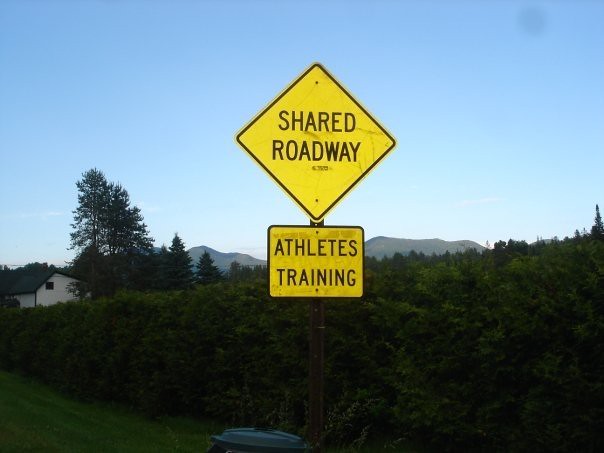This nature-themed photograph captures a picturesque landscape featuring a harmonious blend of natural and man-made elements. In the foreground, a weathered gold roadside sign with black text reading "Shared Roadway Athletes Training" is prominently displayed on a post. The sign has a slightly dirty, grayish appearance and stands next to a green circular object. Behind the sign, dense green shrubbery and bushes intersperse with patches of vibrant green grass.

To the left of the sign, a charming white house with a contrasting black roof nestles amid several tall trees. The backdrop is dominated by a range of majestic mountains, their peaks standing proudly under a stunningly clear blue sky with barely a cloud in sight. The image quality is exceptional, capturing every detail crisply and vividly, offering a serene and detailed snapshot of this tranquil setting.